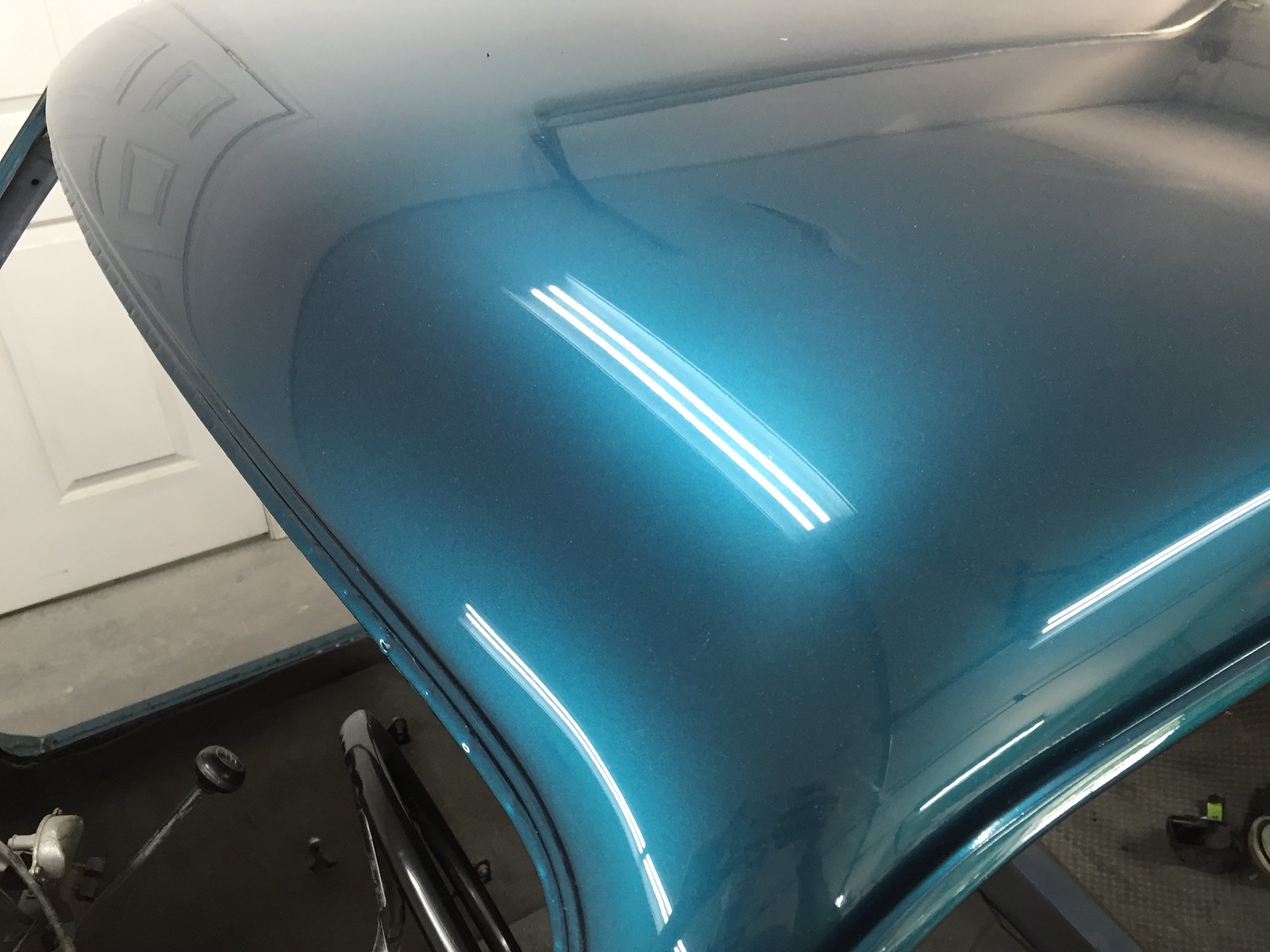This image depicts a close-up view from above of a metallic blue vehicle, possibly a car or a golf cart, showcasing a shimmering, lighter blue rooftop. The vehicle notably lacks glass windows, windshields, and doors, revealing the black interior components—a black steering wheel and a rounded black stick shift attached to a silver rod. Illuminating the front part of the roof is a set of fluorescent track lights in a white and blue housing. Visible reflections on the roof suggest the scene is set inside a garage, with the reflections capturing both the white walls and the rail of the garage door. The cement floor of the garage is clearly visible, and in the background, there is a distinctive white door with a squared pattern indented into it.